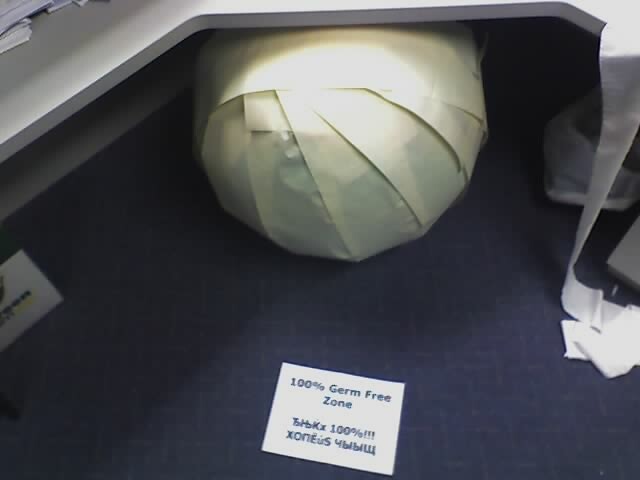The photograph depicts a scene from what appears to be an office or cubicle. Dominating the foreground is a ball—possibly an exercise ball—wrapped meticulously in what seems to be white or cream-colored toilet paper, a shade influenced by the lighting. The ball is situated underneath a light gray, hexagon-cutout countertop. In front of the ball, there's a white card with blue lettering prominently displaying "100% germ-free zone" in English, alongside additional text in multiple languages.

The office space features a blue carpeted floor and a cluttered stack of papers is visible in the top-left corner of the image. On the right side of the desk, a roll of unfurled toilet paper extends to the floor, next to a trash bin containing a white bag. The entire setup suggests a humorous prank or an exaggerated attempt to maintain cleanliness, with the ball wrapped up, possibly as a measure to stay germ-free.